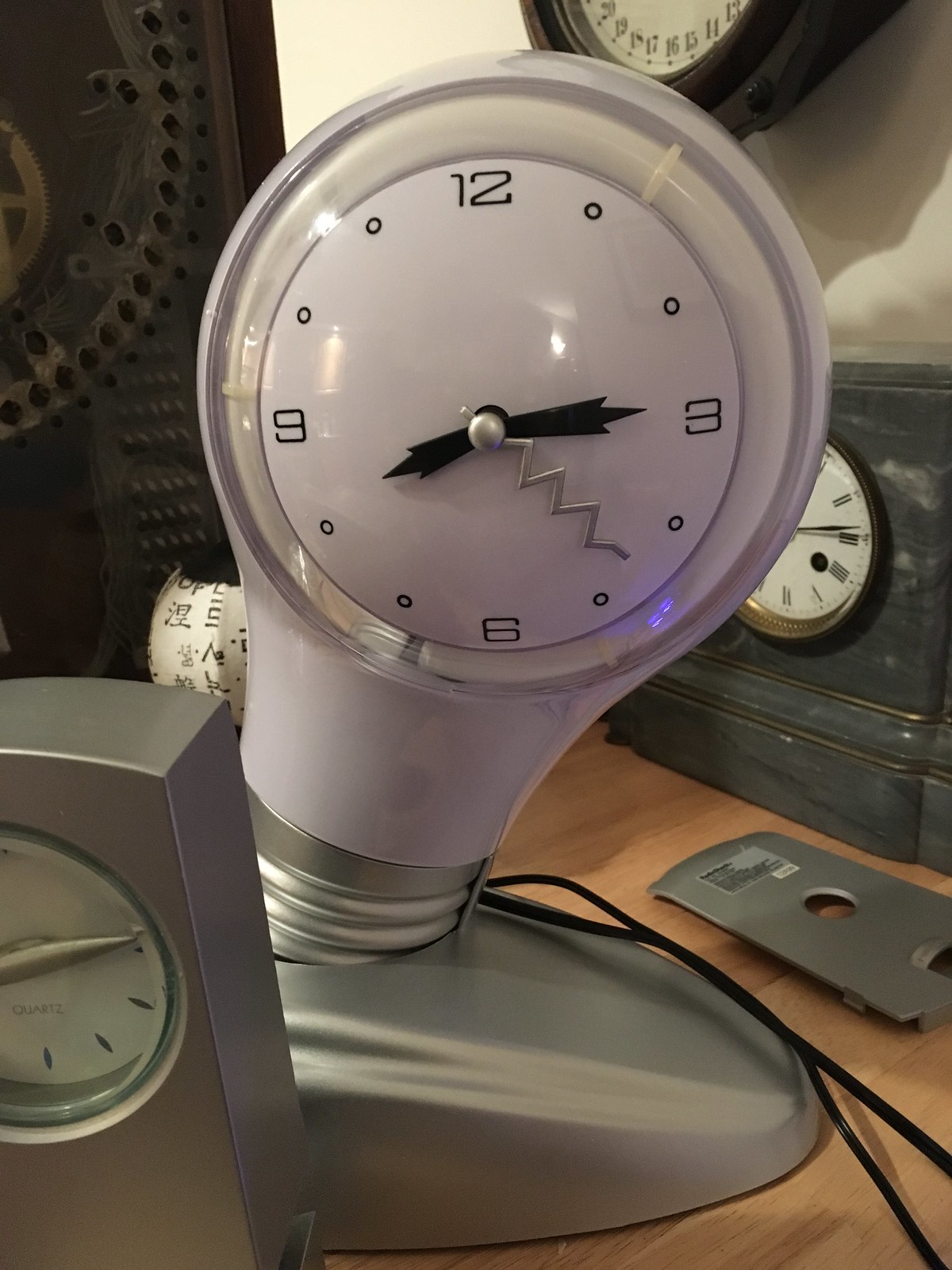The image features a collection of uniquely designed clocks centered around a fascinating clock shaped like a light bulb. The main focus is a light bulb-shaped clock set on a light brown wooden tabletop. This clock has a large oval silver base resembling the screw end of a light bulb, a white clock face displaying only the numbers 3, 6, 9, and 12, black hour and minute hands, and a distinctive squiggly silver seconds hand.

To the bottom left of the image, there is a small rectangular clock with a silver-handed mechanism visible through a glass window. This clock has a white face but no numbers, adding to its minimalistic design.

In the back right, partly obscured, is a gray stone-style clock. Its dial is white, with Roman numerals marking the hours, and it features a golden circular rim around the clock face.

The overall composition highlights the variety and creativity in clock design, anchored by the striking light bulb-shaped clock at its center.